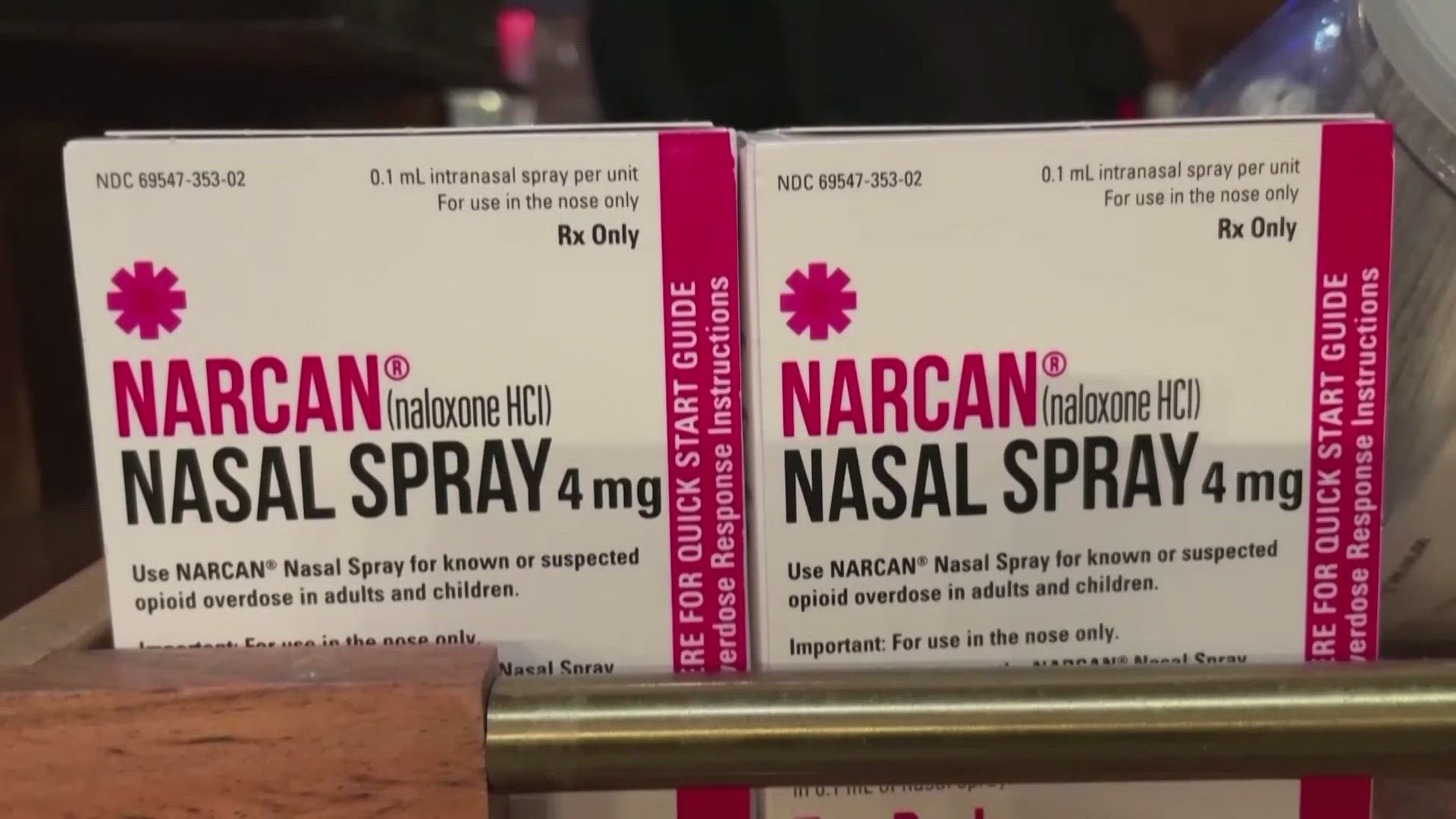A rectangular horizontal photograph captures two identical informational booklets for Narcan nasal spray displayed alongside each other on a wooden and brass metal bookshelf. Both white booklets feature a prominent dark pink line on the right-hand side, with "Quick Start Guide and Response Instructions" written in white letters. A brass bar partially obscures some lettering on the package fronts. On the left side, below a pink starburst, the bolded word "Narcan" with a registered trademark symbol stands out in pink lettering. Immediately to the right in black text, it reads "Naloxone HCl," and below that in bold black letters, "Nasal Spray 4mg." Additional smaller black text appears beneath it. The top right corner of each booklet states "Rx only" and specifies "1.1 ml intranasal spray per unit" for use in treating known or suspected opioid overdoses in adults and children, emphasizing that it is for intranasal use only.